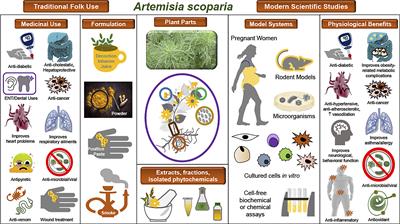The image is a low-resolution informational chart titled "Artemisia Scorparia," featuring both traditional folk use and modern scientific studies. The chart is divided into multiple readable columns labeled "Medicinal Use," "Formulation," "Plant Parts," "Model Systems," and "Physiological Benefits." It includes various images with blurry black labels, showing graphics of someone squeezing something from a tube onto their finger, a pair of lungs, and a tired-looking individual. The visual elements are presented in a spectrum of colors including browns, yellows, greens, reds, grays, blues, and whites. The poster aims to juxtapose traditional applications of Artemisia Scorparia against its scientifically studied benefits, illustrating its effects on different parts of the body, potentially for treating various medical conditions.